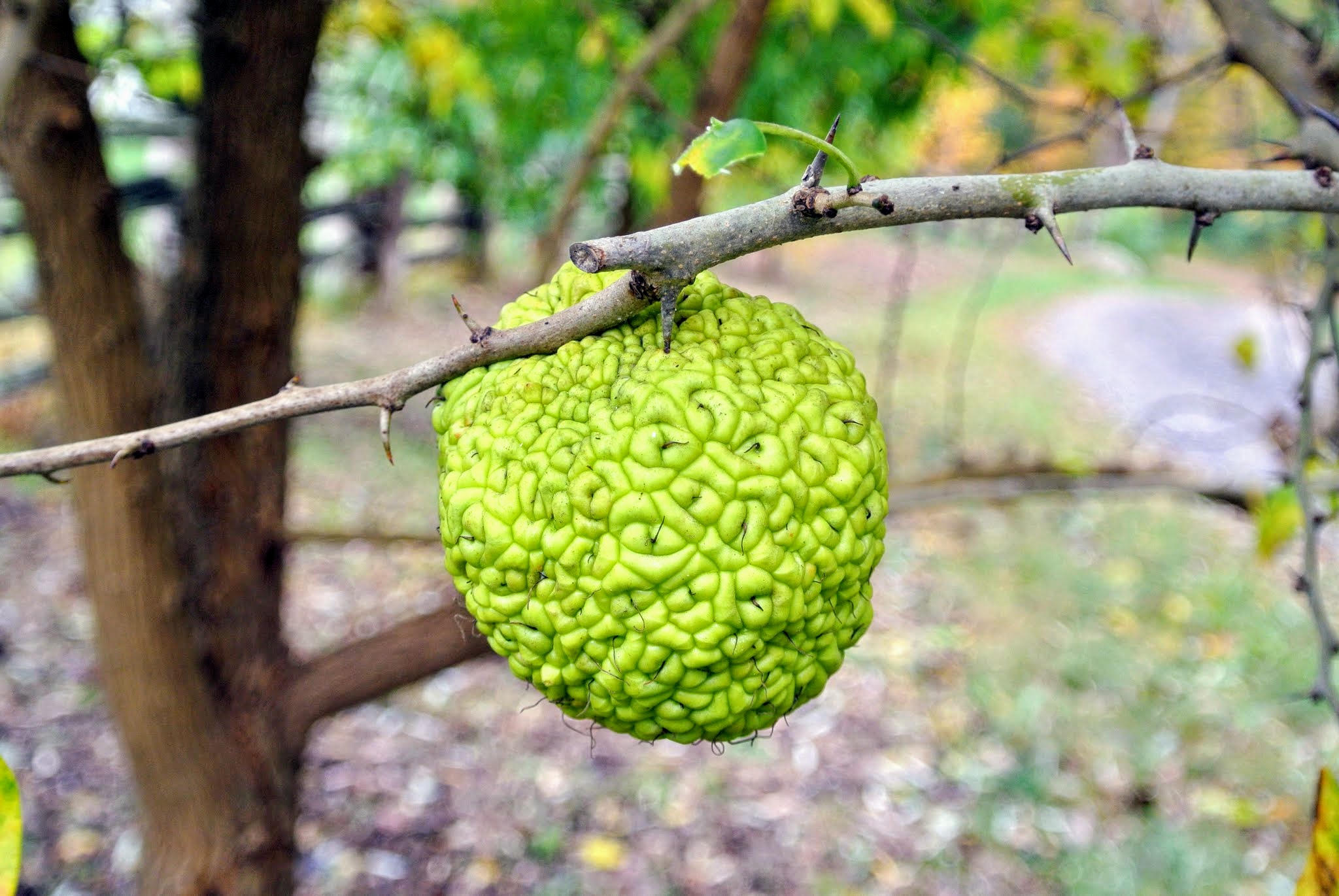This photograph captures a bright yellow-green, tennis ball-sized fruit distinctively textured like reptile skin or brain-like segments, hanging from a partly-pruned, aged branch covered with roughly 12 thorns and a touch of moss. The fruit, which appears inedible and very rigid, exhibits small hair-like structures at its base. Surrounding the focal point with the fruit, the background fades into a soft blur revealing a natural outdoor setting with overlapping scenes of green and yellow foliage, a grassy ground, a potential cement path, and additional trees, all bathed in daylight, creating an abstract yet harmonious landscape.